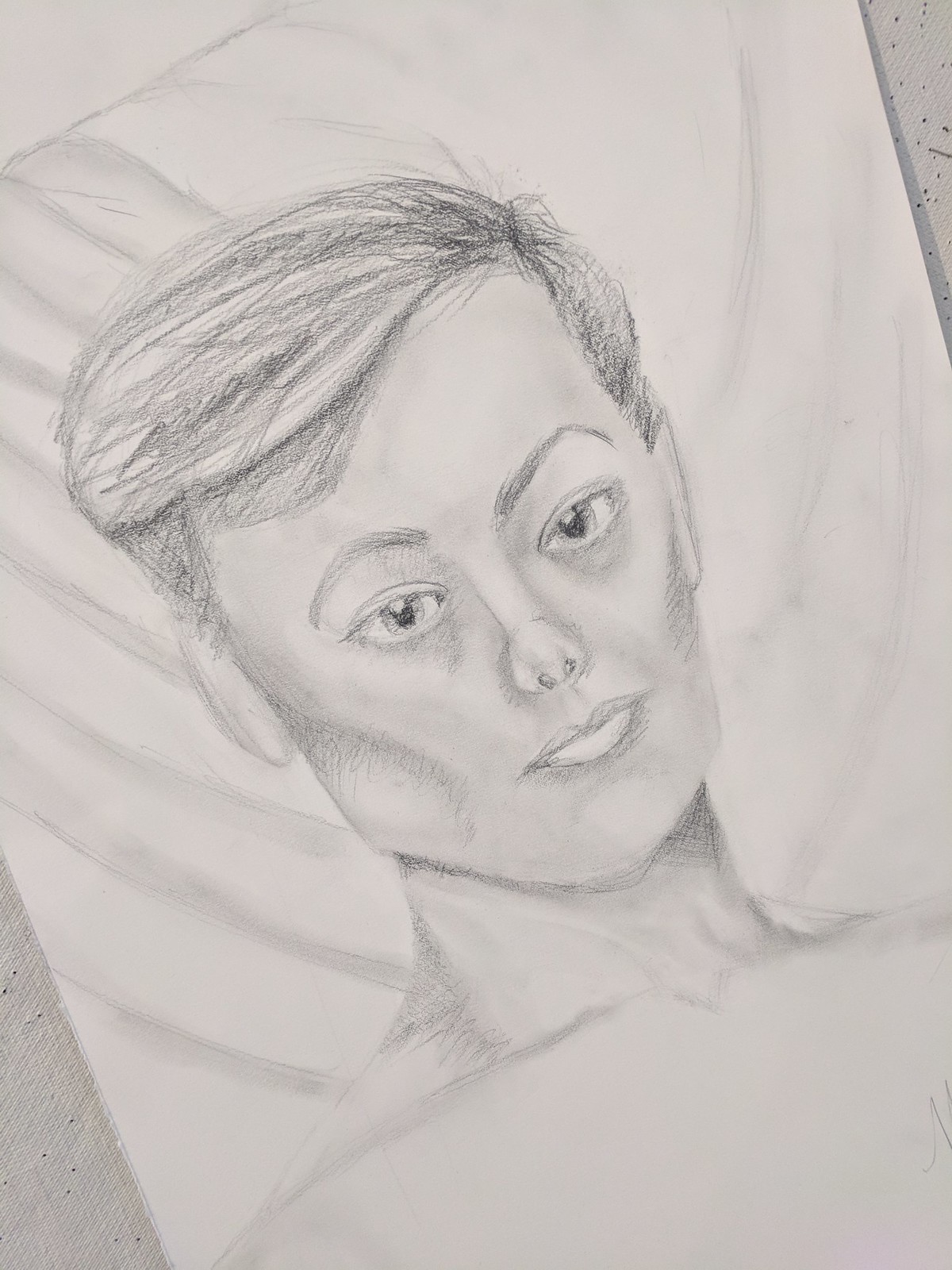This is a detailed pencil sketch of an individual drawn on a tan-like paper, utilizing a grayscale color palette. The portrait, possibly using charcoal or a similar medium, depicts a person with a strong and angular face, featuring defined cheekbones. Their hair is parted from the left side to the right, with the part itself visible on the right side of the image. The eyebrows are high-arched, and the eyes are highly detailed, featuring reflective highlights that lend an inviting expression. The nose is delicately shaded, with a small, upturned tip that offers a glimpse into the nostrils. Their lips are average in size yet slightly pursed, giving a narrow appearance to the mouth. The chin is strong, contributing to a youthful look, and the neck is similarly strong, supported by broad shoulders that are partially visible. Behind the head, draped lines suggest the presence of fabric, perhaps a pillow or a curtain, adding depth to the portrait. The sketch, rich in shading and detail, captures a striking and expressive likeness of the individual.